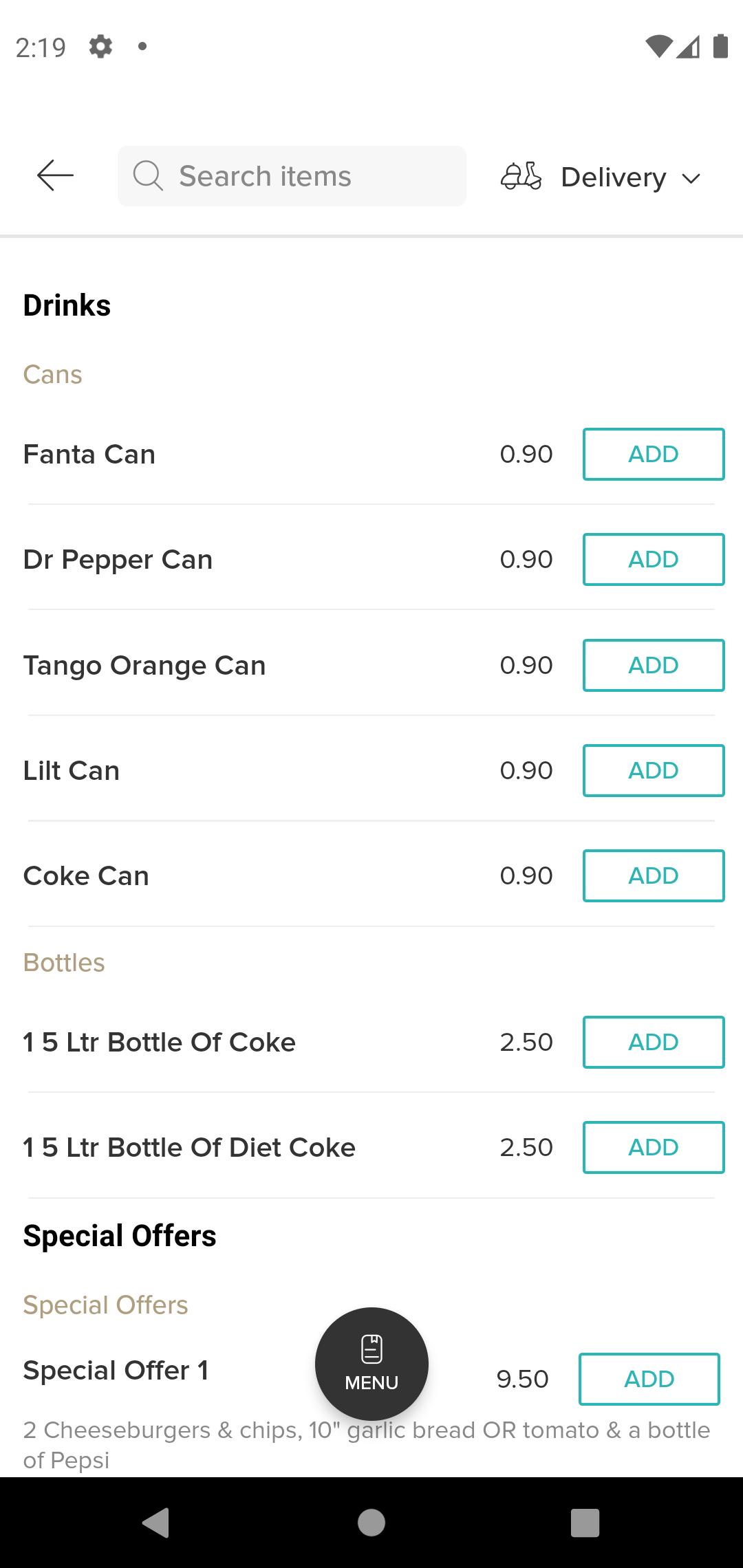Screenshot of a food delivery service app showcasing the beverage selection page. At the top of the screen, there's a search bar labeled "Search Items." Below the search bar, the page is categorized into different sections: "Drinks," followed by "Cans," listing various sodas. Each can, including Fanta, Dr. Pepper, Tango Orange, Lilt, and Coke, is priced at 90 cents, with an "Add" button next to each.

Further down, there's a "Bottles" section listing 1.5-liter bottles of Coke and Diet Coke, both priced at $2.50. The page also highlights a "Special Offers" section with an item priced at $9.50. 

The layout is user-friendly, aiming to facilitate easy navigation and quick choices for the user.